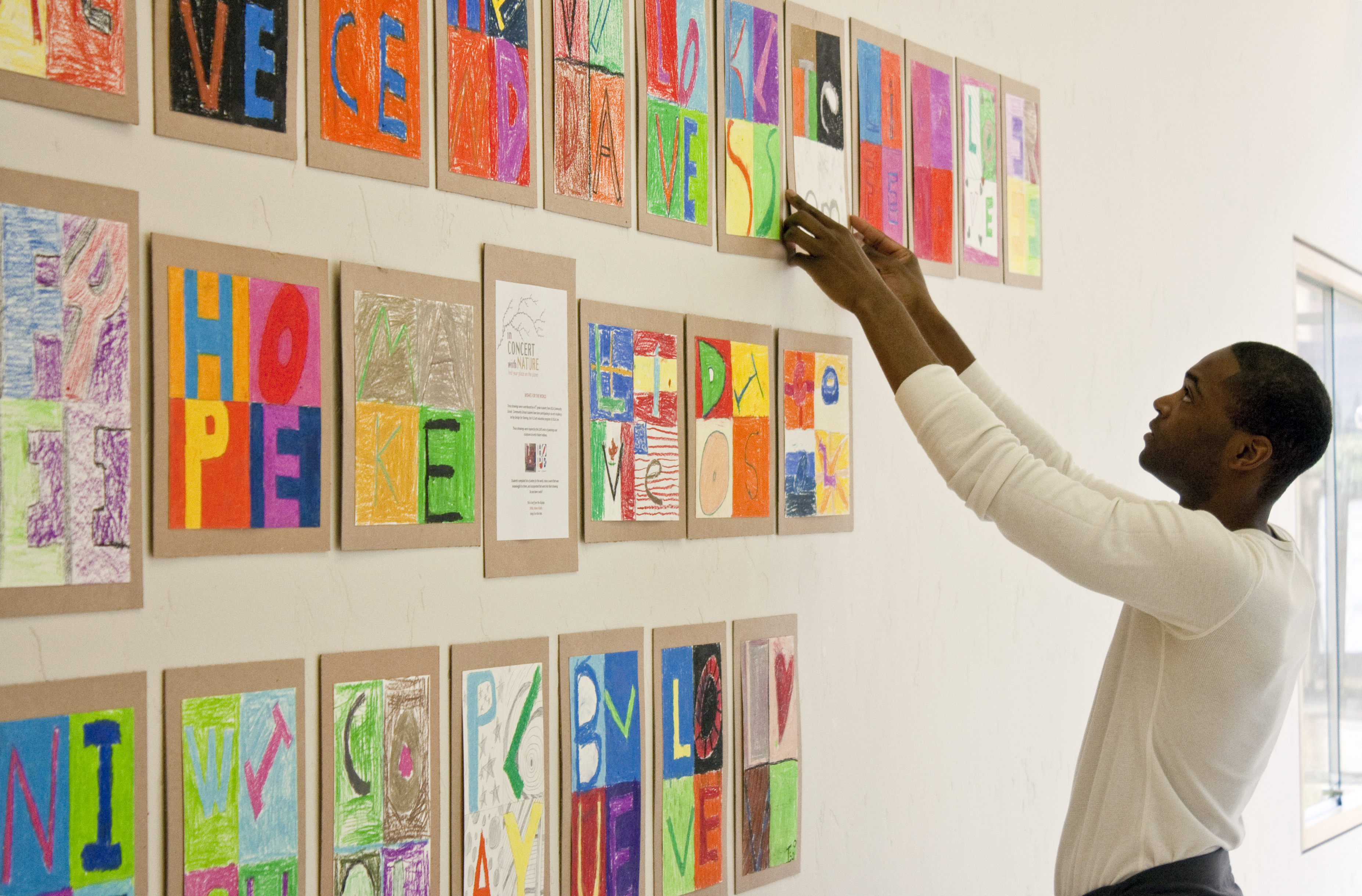The image features an African-American man, wearing a thin, long-sleeved white shirt and black pants, standing in front of a white wall. He has neatly cut hair and is seen reaching upwards, adjusting or hanging a piece of artwork. The wall displays three neatly arranged rows of vibrant artwork that appear to be homemade, possibly created by children. Each piece of art, crafted on segments of cardboard with colored paper, contains bright and diverse colors including blue, orange, purple, red, pink, yellow, white, and black. Many of the artworks include words like "hope," "love," "kindness," and "play," arranged in four squares each. The environment is filled with natural light, with hints of a glass door or screen in the background, contributing to a bright and vibrant setting. The clear image suggests the man may be a schoolteacher, carefully ensuring the children's artwork is straight and in order on the wall.